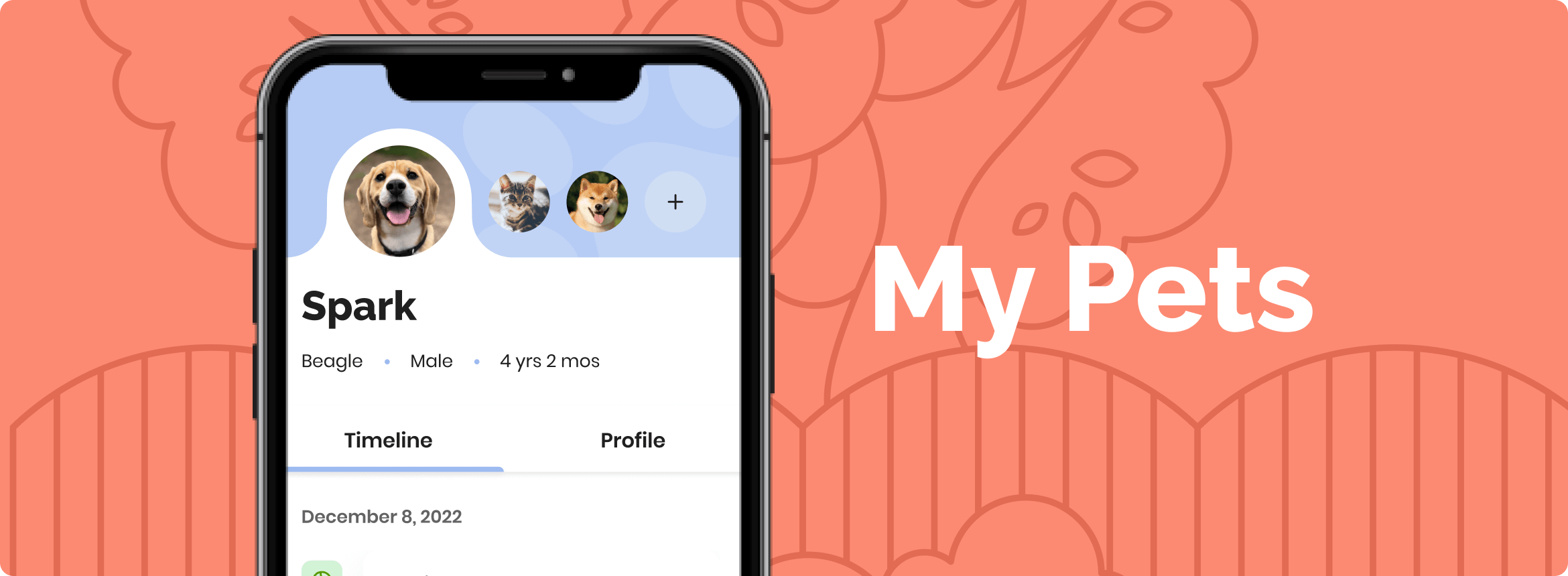In the center of the image, a partially visible smartphone screen stands out against a vibrant, animated background dominated by a coral-peach hue. The background features stylized trees, a fence, and bushes all rendered in this peach color, adding a whimsical touch to the scene. 

The smartphone, with a silver and black frame, displays a periwinkle-colored header. The main focus on the screen is a tab featuring a brown and white Beagle dog with a black nose and a pink tongue hanging out. The dog's profile text, displayed in black, identifies him as "Spark," a 4-year-2-month-old male Beagle. Beneath the dog’s name, the text "Timeline" is highlighted, followed by an underline, and next to it, the word "Profile" is visible. Just below this header, the date "December 8, 2022" appears in gray text.

To the right of Spark's profile, two additional images are partially visible. One shows a gray cat, while the other features another dog with a coat that gradates from brownish-beige at the ears to white towards the mouth area, with the ears being the darkest part.